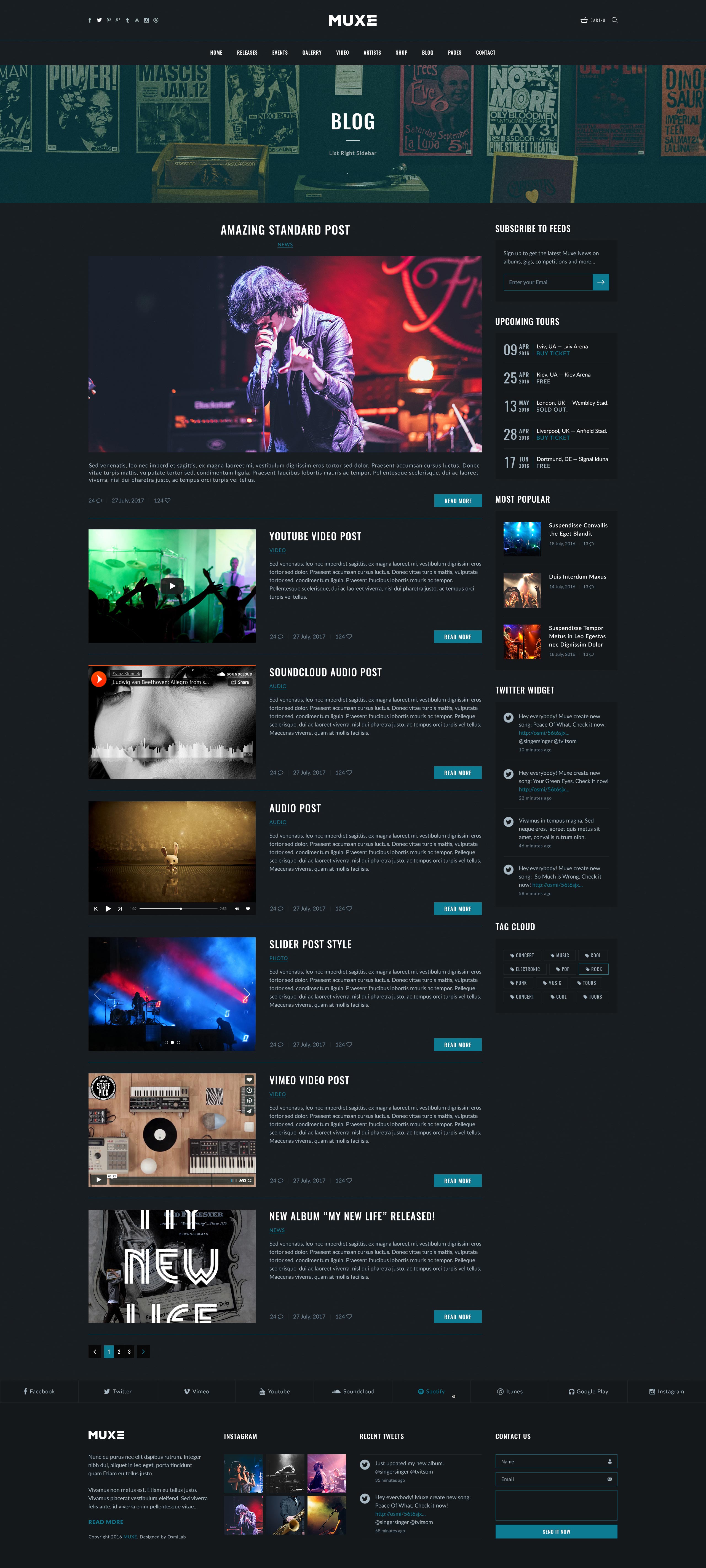This is a color image predominantly featuring black with white text accents and several dark-toned photographs. It showcases a mock-up of a website named "Muxe" (M-U-X-E), dedicated to music. Across the top of the website, a banner menu displays various tabs including Home, Releases, Events, Gallery, Video, Artists, Shop, Blog, Pages, and Contact. The specific page shown in the image is the Blog section.

In the center, a photo of a male rock musician donning a leather jacket is prominently featured. He has long black hair that obscures his eyes and stands at a microphone, emoting passionately while extending his left hand. To the right of his image, a text box labeled "Upcoming Tours" lists several tour dates and locations such as Lviv, UA (Ukraine), various cities in the UK, and Dortmund, DE (Germany).

Beneath the tour information, there are sections for feeds or articles that users can subscribe to or read further. These include a YouTube post and a SoundCloud audio post, each accompanied by music-related thumbnail images. Examples of these thumbnails include a concert scene, a close-up of the singer's face, and a conceptual album cover featuring a toy bunny rabbit.

Of note is that all small text on the website consists of lorem ipsum — placeholder text commonly used in printing and typesetting — which serves as a visual filler. Headlines like "Twitter Widget" appear, but the detailed content is in Latin dummy text, indicating that the site is still in the mock-up stage.